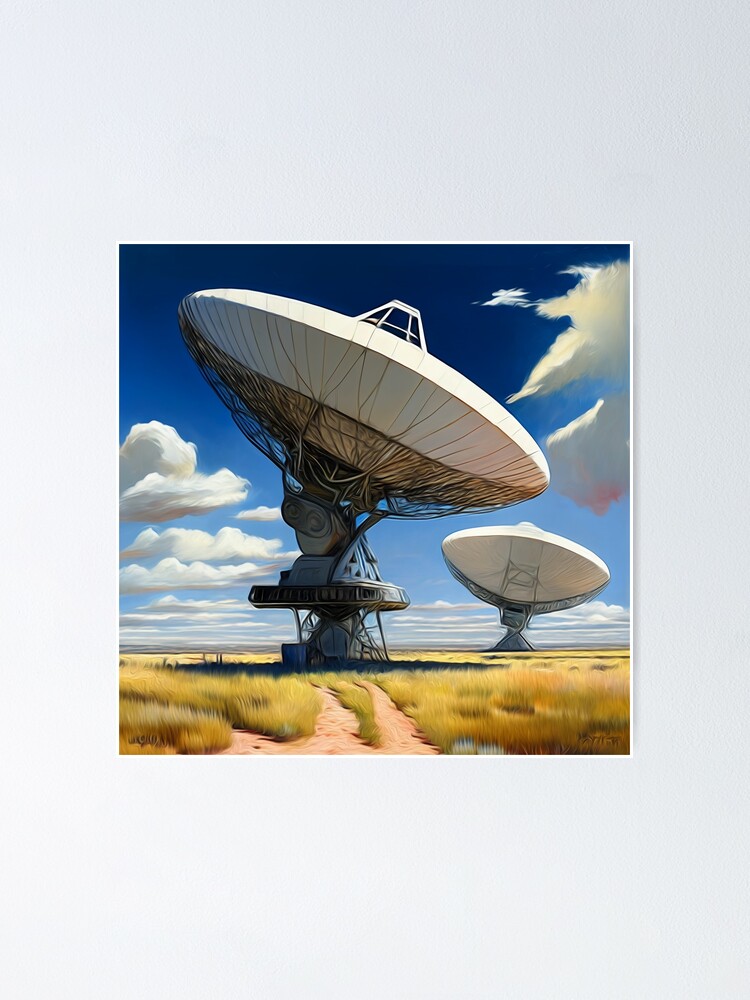The image is a highly stylized, semi-photorealistic painting that, at first glance, appears to be a photograph. It depicts an outdoor scene with a bright blue sky adorned with fluffy clouds both in the foreground and distant background. Dominating the immediate foreground is a large, white, circular radio telescope or satellite antenna, characterized by numerous gray cables extending to an irregularly shaped silver metallic base. A dirt road leads up to this main telescope, passing through patches of yellowish-green grass.

Further into the background, to the far right of the image, there is another identical radio telescope, slightly smaller and partially obscured by the distance. The painting captures the sunlight gleaming off the metallic surfaces of the telescopes, casting subtle reflections and shadows, indicating it's around noon. The expansive open field under the cloud-streaked sky and the meticulous detail in the landscape contribute to the serene, isolated feel of the scene. The painting is rendered with an acrylic technique, bordered in thin white and mounted on a gray background, enhancing its presentation as an art piece.